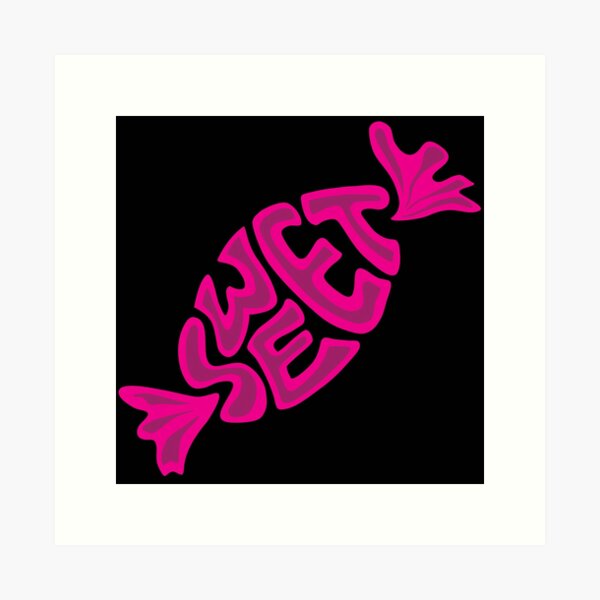The image features a central design that appears to be digitally created, possibly hand-crafted as well, featuring a distinctive layering of borders and colors. At the outermost perimeter is a light gray rectangle, which frames a thick-bordered white square. Inside this white square is a solid black square, perfectly centered. Dominating the center of this composition is a logo crafted in a dark pink hue. This logo, set against the black background, spells the word "SWEET" in an unconventional fashion—diagonally from the bottom left to the top right. The letters are arranged creatively: S is at the beginning, followed by W above E on the second line, another larger E to the right, and finally T at the end. Completing the design are wing-like or green stem-like shapes adorning the lower left and upper right corners of the letter formation, giving it a playful, slightly feminine or girly aesthetic. The meticulous arrangement and the specific colors of off-white, eggshell white, black, pink, and dark pink contribute to a visually striking and balanced piece.